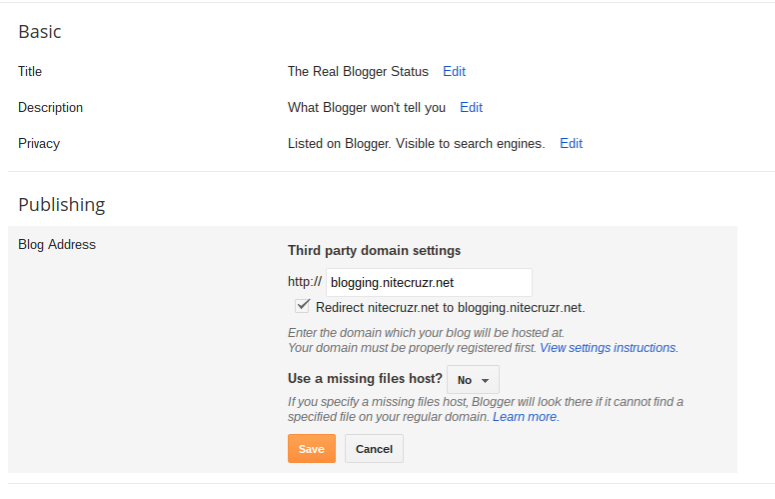Here's a refined and detailed caption for the image described:

---

"Screenshot of a Blogger settings page with a clean white background, primarily featuring black and gray text, interspersed with blue and orange elements. The title at the top reads 'Basic.' Below it, the section header 'Title' is followed by the phrase 'The Real Blogger Status' with an 'Edit' option in blue text.

The next section is marked 'Description,' containing the phrase 'What Blogger won't tell you,' again with an 'Edit' option in blue. Further down, the 'Privacy' section notes that the blog is 'Listed on Blogger' and 'Visible to search engines,' accompanied by another blue 'Edit' link.

A gray horizontal line divides the page, leading to the 'Publishing' section. Here, a large gray box is labeled 'Blog Address,' beside which the 'Third-party Domain Settings' feature an entry field with 'http://blogging.nightcruiser.net.' This URL is enclosed in a white text box.

Below this, a checkbox is labeled 'Redirect nightcruiser.net to blogging.nightcruiser.net.' An informative note follows: 'Enter the domain which your blog will be hosted at. Your domain must be properly registered first. View settings instructions.'

Further down, the page addresses 'Using a missing files host,' currently set to 'No.' It explains that 'If you specify a missing files host, Blogger will look there if it cannot find a specified file on your regular domain,' with a 'Learn more' link in blue text.

At the bottom of the page, there are two buttons: a white and orange 'Save' button and a black and gray 'Cancel' button."

---

This detailed caption captures the specific elements and layout of the described screenshot, enhancing understanding without altering the original content.